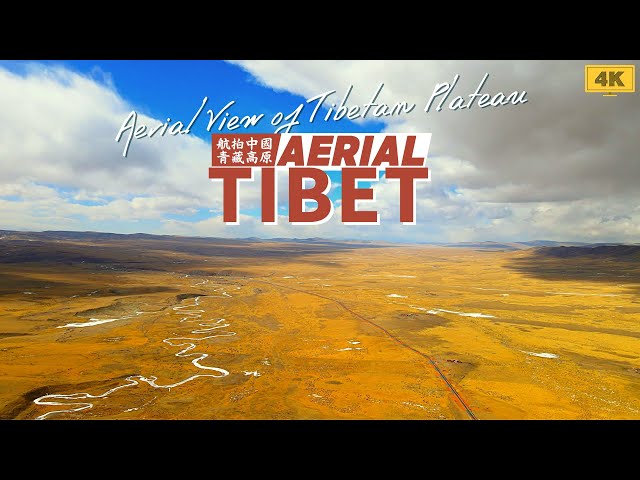The image is an aerial view of the Tibetan Plateau, captured in a high-resolution 4K format, as indicated by the "4K" text in the upper left corner. The top and bottom of the image feature solid black bars, enhancing the focus on the central content. Across the top, slightly slanted, the text "Aerial View of Tibetan Plateau" is prominently displayed in white, underlined by a red logo with "Aerial Tibet" in white outline. Adjacent to this text are Chinese characters in a red box. The day is sunny with a bright blue sky dotted with patches of flat white and gray clouds, casting shadows on the ground below. The plateau itself is a vast, barren expanse of brown to light brown earth, marked by dry riverbeds and a dark line that possibly denotes a road stretching towards the horizon. In the distant background, the landscape features faint ridges that may be mountains. There is no visible wildlife or vegetation, underscoring the stark and arid beauty of the region.